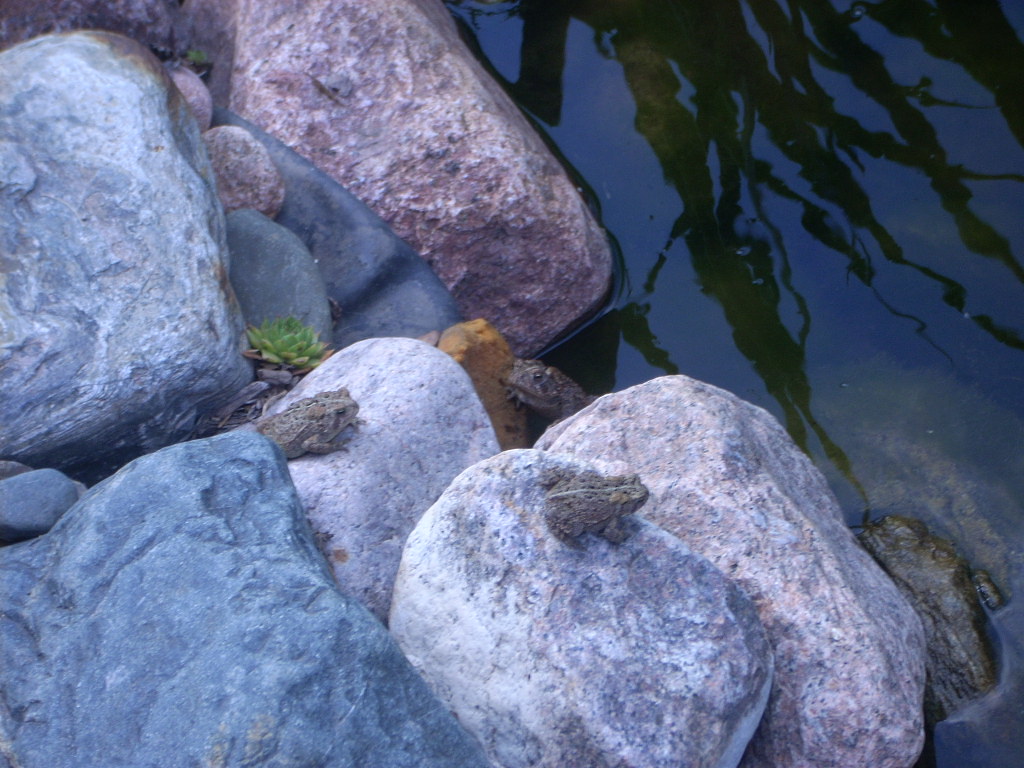The image depicts a serene pond area dominated by large, stacked rocks in varying shades of gray, tan, and hints of purple and yellow. The water, primarily situated on the right side of the image, appears dark and murky, partially due to shadows and green algae. Reflections of tall plants with elongated leaves can be seen across the water's surface. Within this natural setting, three medium-sized frogs with textured, rough skins in dark green-brown hues blend seamlessly into their rocky environment. Two of the frogs are perched on some of the highest rocks, one seemingly poised to jump, while the other appears more relaxed. The third frog, larger in size, is partially emerging from the water in the corner between the rocks. The overall scene captures a well-camouflaged, tranquil moment in nature.